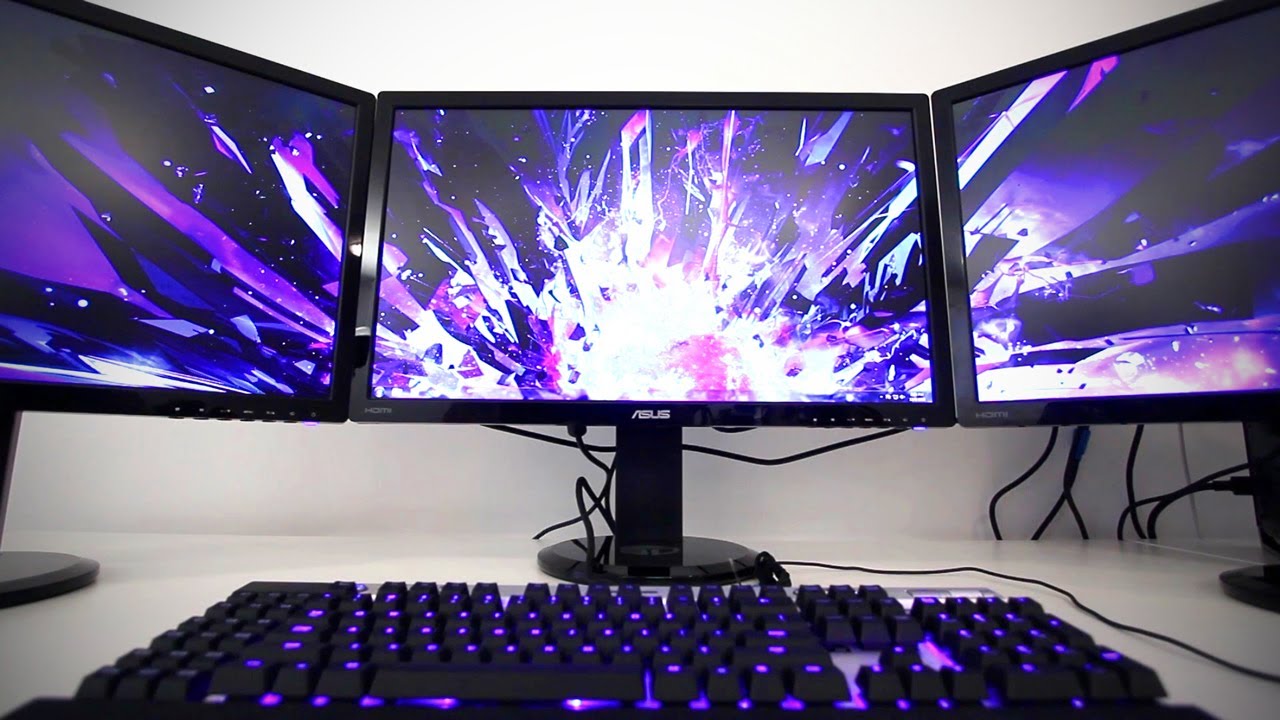In this close-up photograph taken on top of a white desk, we see a sleek black keyboard illuminated with a vibrant neon purple backlight. Dominating the scene is an impressive triple-monitor setup, where three monitors are seamlessly connected side-by-side, presenting a continuous, striking image. The display shows an explosion of fireworks, with a brilliant burst of white light at the center that gradually transitions into shades of light and dark purple, eventually blending into a deep black background. All three monitors are encased in elegant black frames. The center monitor features the brand name "Asus" prominently displayed at the bottom of the screen. Numerous black cords trail down from behind the monitors, disappearing out of view behind the desk, hinting at the technical setup powering this visually captivating workspace.